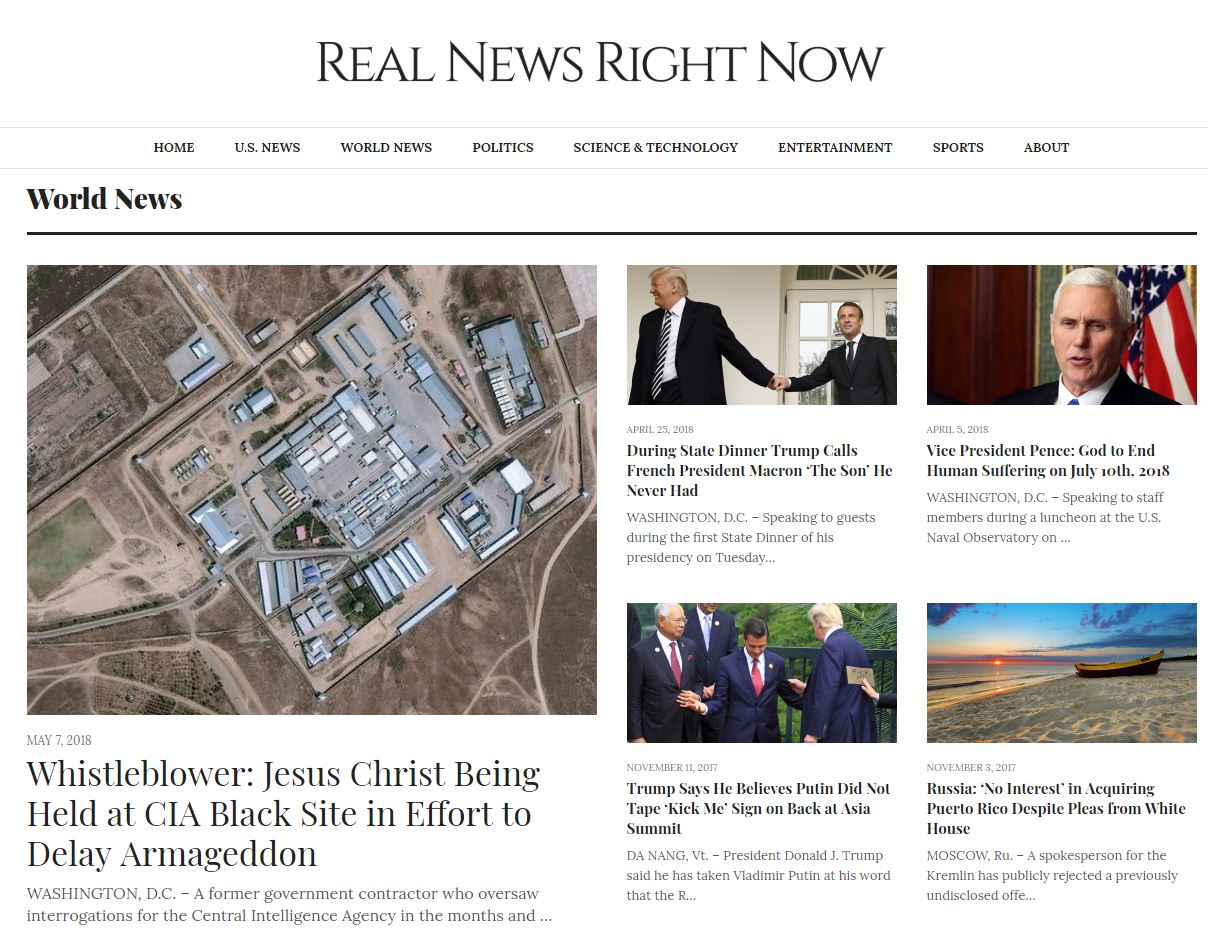This is a screenshot of a news website, identified at the top by a prominent header in big black font reading "Real News Right Now." Below this header is a horizontal navigation bar featuring category options, starting with "Home," followed by "US News," "World News," "Politics," "Science and Technology," "Entertainment," "Sports," and finally "About" positioned at the far right.

The page currently displayed is "World News," as indicated by the section title "World News" placed at the top left of the page, separated from the body of the webpage by a thin black divider line. The main content area features a large thumbnail image of an aerial view of a complex. Below this image is the lead article headline, which reads, "Whistleblower Jesus Christ Being Held at CIA Black Site in Effort to Delay Armageddon," along with the publication date located at the top left of the title.

To the right of this lead article are four additional news stories, each accompanied by smaller thumbnail images. These stories are arranged in a two-by-two grid format, with two articles positioned at the top and two more directly below them.